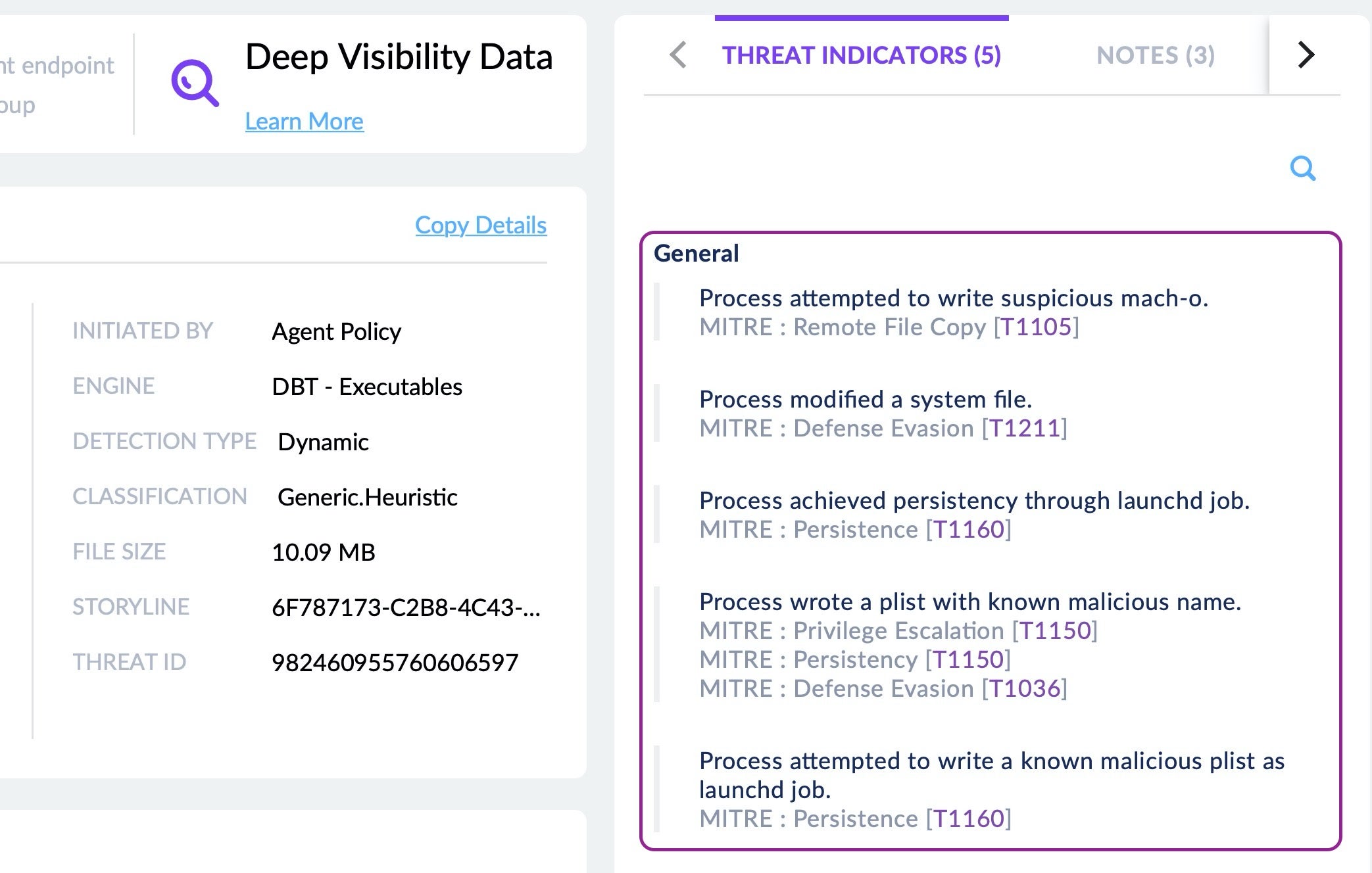In the upper left corner, the header "Deep Visibility Data" is prominently displayed next to a distinctive purple hourglass icon. Below this header, there is a section titled "Copy Details," featuring a text box with detailed information. The text box states that the data was "Initiated by agent policy engine DBT," with the detection type categorized as "Dynamic Classification, Generic Generic Heuristic." The file in question has a size of 10.09 megabytes and the storyline code is "6F787173C2B84C43." Additionally, the threat ID is marked as "982460955760606597."

On the right side of the page, the "Threat Indicators" section, which is highlighted, lists five specific indicators. Under the "General" subheading, several processes are described: 
1. "Process attempted to write suspicious match."
2. "Process modified a system file."
3. "Process achieved persistency through launchd job."
4. "Process wrote a plist with a non-malicious name."
5. "Process attempted to write a non-malicious plist as launchd job."

This detailed display seems to be part of security software, offering a comprehensive overview of detected malicious activities and general system information, showcasing various types of attacks and their respective data for assessment.